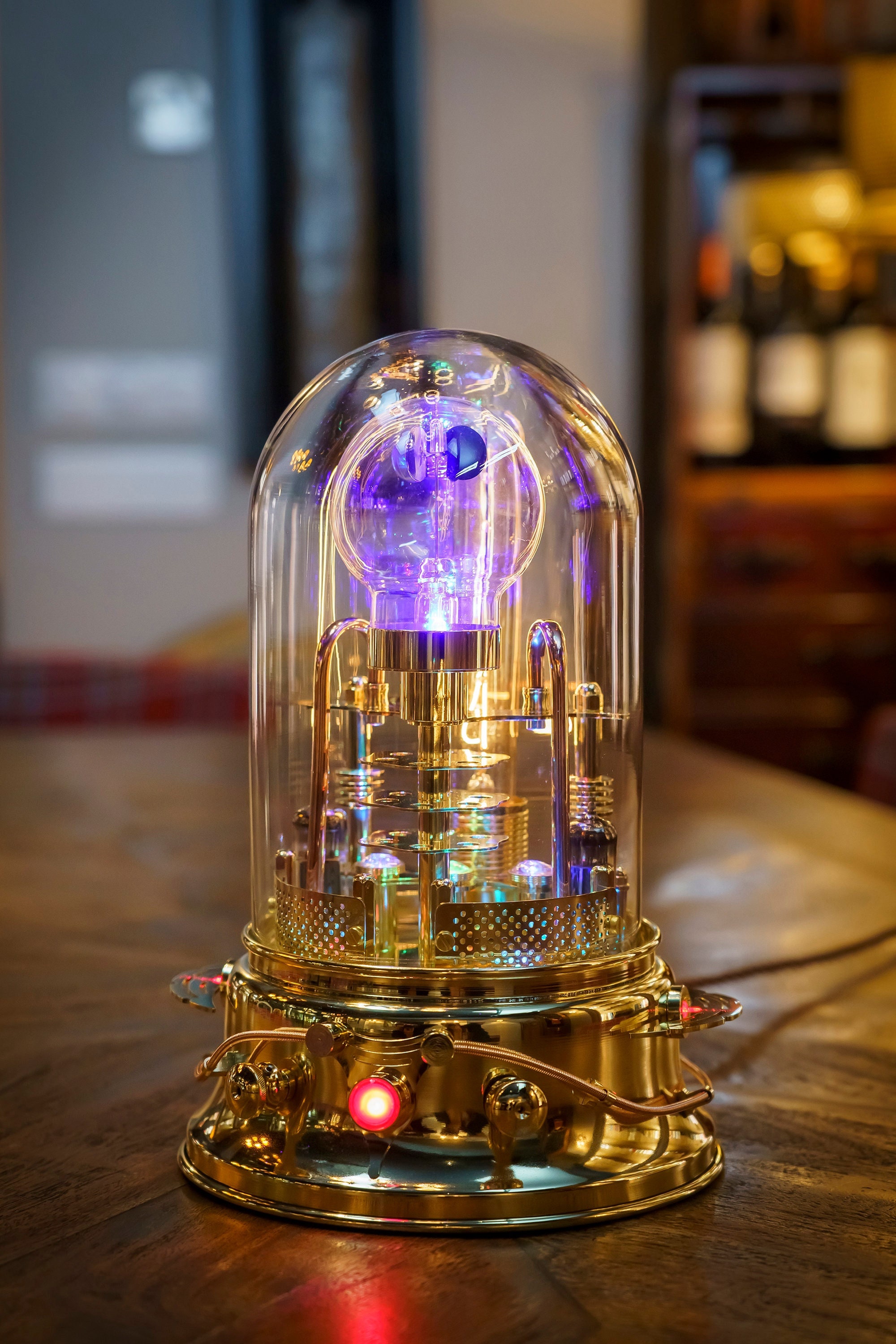This indoor close-up photograph showcases an intricate, modern lighting device that blends elements of a lantern and an electrifying device. The base, made of a golden metal, sits on a brown wooden table and features a distinctive glowing red light at its center, alongside golden wires and knobs. Above the base, a clear glass dome encases more golden tubes and wires, culminating in a unique light bulb at the top that emits a bluish-purple glow, reminiscent of those interactive electric globes. The blurred background reveals a shelf stocked with wine bottles in the upper right corner and a white wall in the back left. This fusion of materials and lighting effects creates a captivating focal point in the scene.